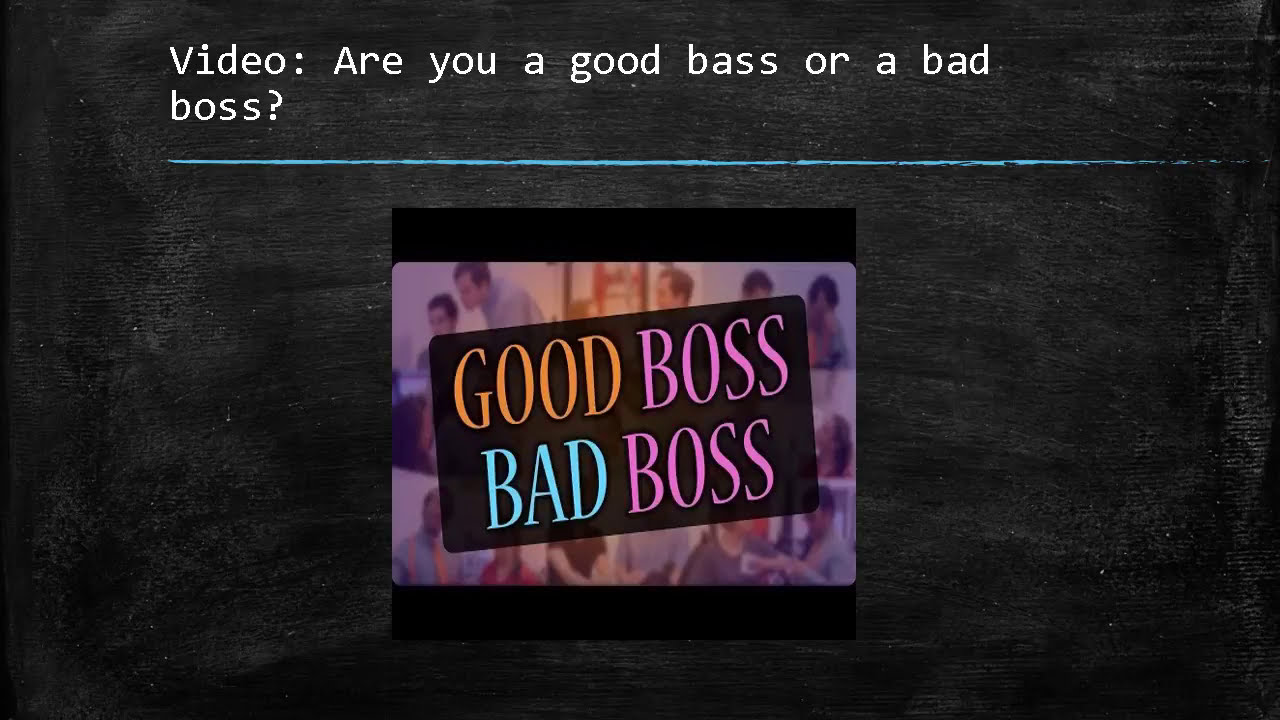The image resembles a PowerPoint slide with a textured black background reminiscent of a chalkboard, lightly speckled with white. At the top, centered white text reads "Video: Are you a good base or a bad boss?", likely containing a typo that should read "good boss". Directly beneath this text runs a thin, light blue horizontal line stretching across the slide. Below the line, there is a central image framed by black borders at the top and bottom. Inside the image, a black rectangle is tilted counterclockwise at approximately a 20-degree angle, featuring the text "good boss, bad boss". The word "good" is in orange, and both instances of "boss" are in light pink, while "bad" is in blue. This text is presented in front of a collage of lightly desaturated photographs portraying office workers interacting, tinted in shades of light purple and gold.